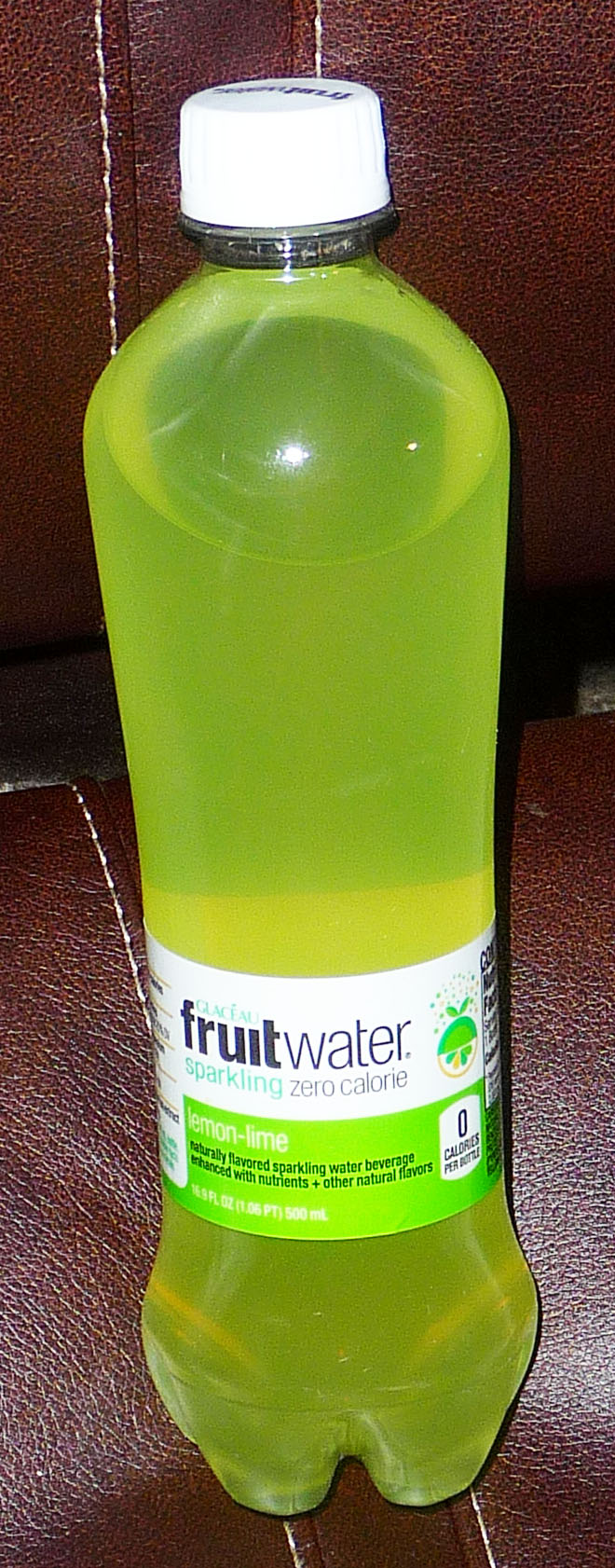This is a close-up photograph of a bottle of fruit-infused water, prominently placed on a stylish car seat. The car seat features luxurious red leather upholstery, meticulously stitched together with white thread, which adds an elegant contrast to the rich red color. The detailed leather stitching is clearly visible due to the extreme proximity of the shot.

The bottle itself is crafted from clear plastic, allowing the vivid green liquid inside to be fully visible. It is topped with a functional white twist cap, designed for easy opening and closing. The label, facing directly towards the camera, proudly displays the text "Fruit Water," along with the descriptor "Sparkling Zero Calorie." This image captures not only the refreshing appeal of the beverage but also hints at a sophisticated lifestyle with its backdrop of high-quality automotive interior.